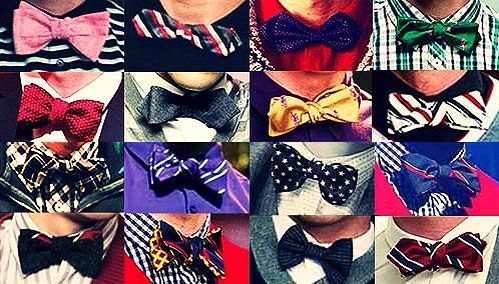This image is a detailed photo grid featuring 16 different bow ties worn by individuals. Each square in the 4x4 grid focuses closely on the neck and upper shirt area of the person wearing the bow tie, showcasing an array of vibrant patterns and colors. Starting from the top left, the bow ties displayed include a pink bow tie, a red and white striped bow tie, a purple sparkly bow tie, and a predominantly green bow tie. The second row features a red sparkly bow tie, a gray bow tie, a yellow bow tie, and a red, white, and black striped bow tie. Moving on to the third row, we see a navy blue bow tie with small white stars, a blue bow tie with white stripes, a green bow tie with white decorations, and a traditional red satin bow tie with polka dots. The last row includes a gold bow tie, a red, white, and blue striped bow tie, a black and white checkered bow tie, and a burgundy bow tie with blue and white stripes. The diverse collection highlights various styles, from traditional to contemporary, in a visually engaging layout.